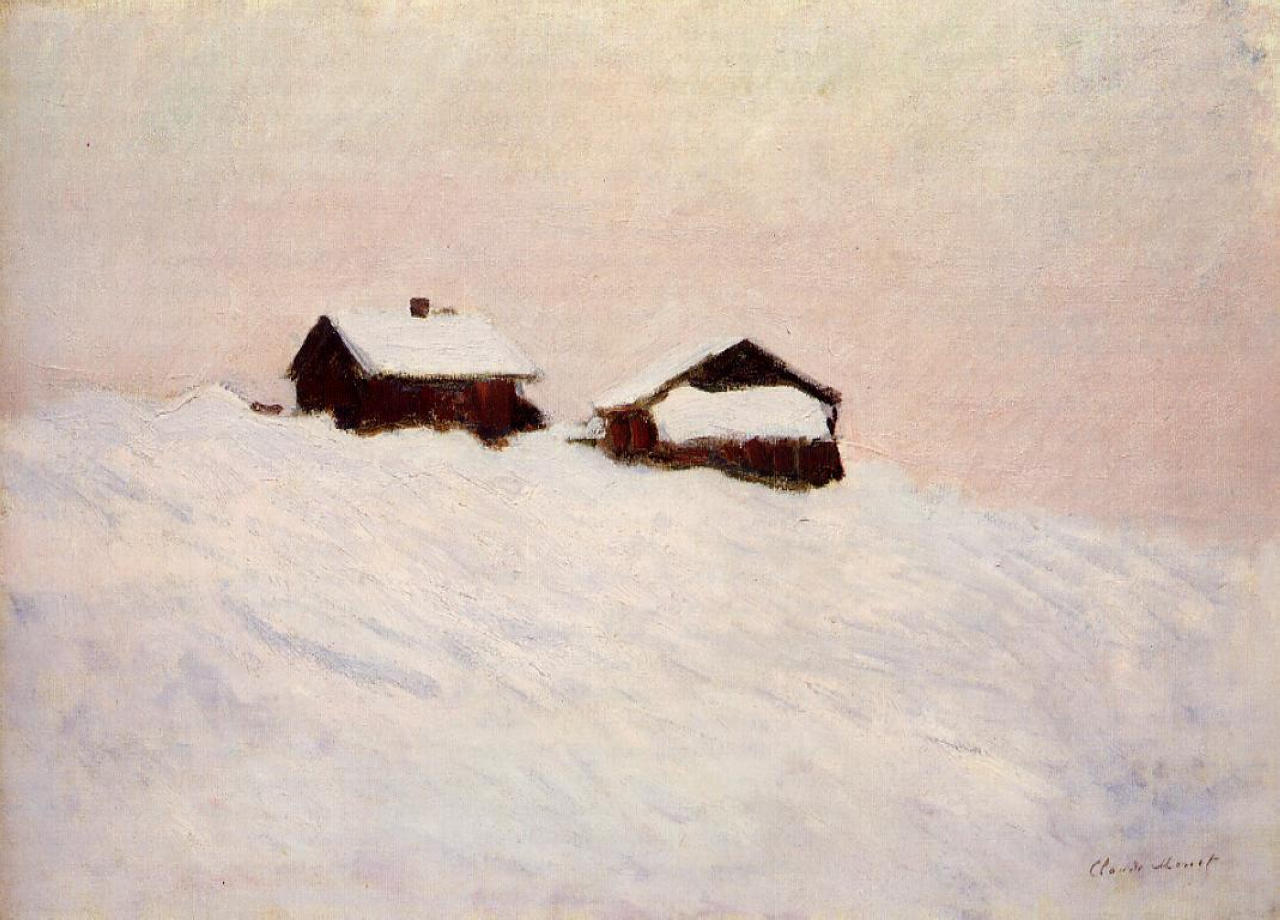This piece of artwork, possibly by Claude Monet judging by the faint signature in the bottom right corner, depicts a tranquil snowy landscape. Central to the painting are two rustic log cabins, dark brown with snow-covered triangular roofs, blending harmoniously against a serene backdrop. The left cabin features a visible chimney, adding to the quaint charm. The scene is set on a textured surface, where the foreground is dominated by layers of white and faint gray snow that convey different depths on what appears to be a sloped terrain or mountain. The sky above transitions softly from pink to subtle hints of gray, with smudged touches of yellow near the top, capturing the diffuse light often seen in overcast or twilight winter scenes. The contrast between the dark brown cabins and the ethereal tones of the snowy landscape and sky creates a captivating and serene imagery, showcasing the tranquility of a winter's day.